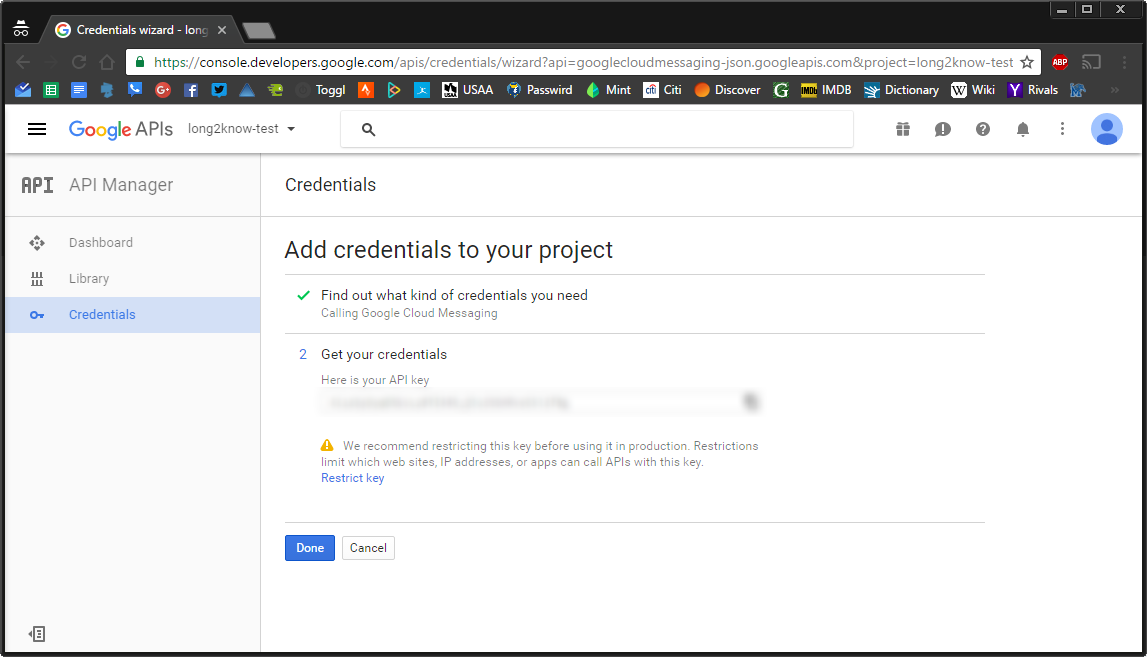The image depicts a web browser window displaying the Google Cloud Console. The top part of the browser features a black header with an Incognito Mode icon on the left, which consists of white glasses and a white hat. The black tab contains a white circle with the colorful Google logo (red, yellow, green, and blue) beside the title "Credentials Wizard - Log" and an "X" for closing the tab.

Below the header, the browser’s address bar displays a green lock symbol followed by "https://console.developers.google.com" in black text, indicating that the connection is secure. Underneath, the main content area of the page is white, and the left side features a menu with three horizontal lines, labeled "Google APIs" in gray.

In the main section, there is a search bar with a black magnifying glass icon. On the right side, the interface shows several icons: a grey gift box with a white exclamation mark, a grey circle with a white question mark, a grey bell, and a series of grey dots. Additionally, there is a blue circle with a white silhouette of a person indicating the user's profile.

The page title "Credentials" is followed by an instruction to "Add credentials to your project." A green check mark and text explain that you need to find out the type of credentials required, suggesting using Google Cloud Messenger to obtain them. Below this, an API key field is presented, but the key is blurred out for privacy.

A yellow rectangle with a white exclamation point highlights a recommendation to restrict the key before using it in production. It mentions that restrictions limit which websites, IP addresses, or apps can call APIs with the key. A blue "Restrict Key" button is available for users to apply these restrictions.